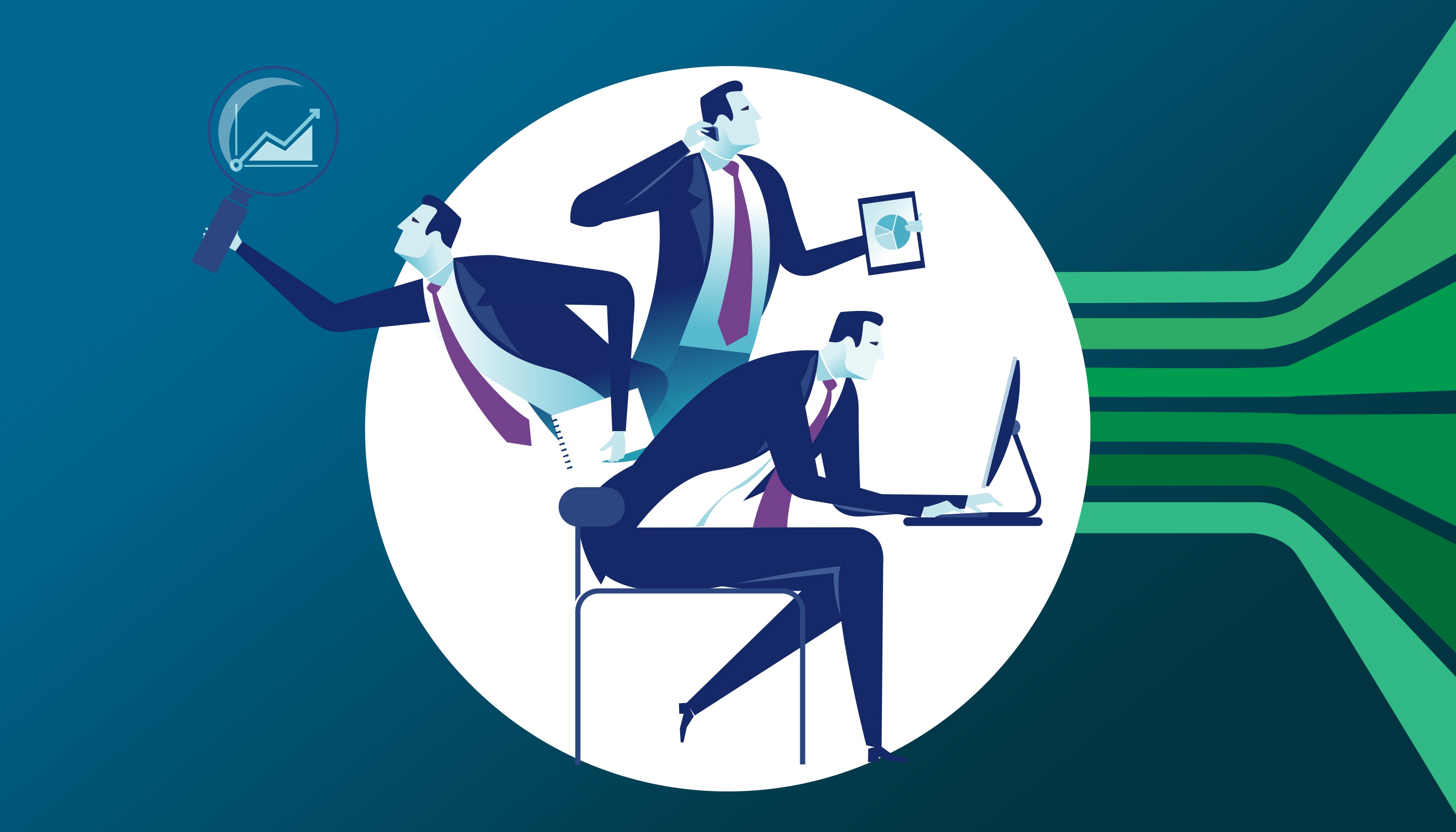This is a digitally animated, horizontal image with a gradient blue background that fades from light blue on the left to darker blue on the right. Extending from the center right side are six green stripes in various shades. These stripes run horizontally before curving as if they have encountered a corner and then fan out toward the top and bottom edges of the image. Positioned centrally is a white circular element. Inside this circle are three images of a businessman, all depicting the same man in different poses. He has black hair and white skin, appears to be in his 20s to 40s, and is dressed in a black suit with a cranberry-colored tie. 

In the center foreground, the man is seated on a wire-framed chair, leaning forward and actively working on an older style silhouette of an Apple computer. Directly behind this seated figure, another portrayal of the same man can be seen standing in profile, with his right arm raised to his ear as if talking on a cell phone and his left arm extended holding a tablet that reveals an image of the Earth. To the left, the third depiction shows the man from the waist up, leaning slightly forward, with his left hand resting by his hip, and his right arm extended outward holding a large magnifying glass, through which a graph appears to be visible. There is no text in the image.